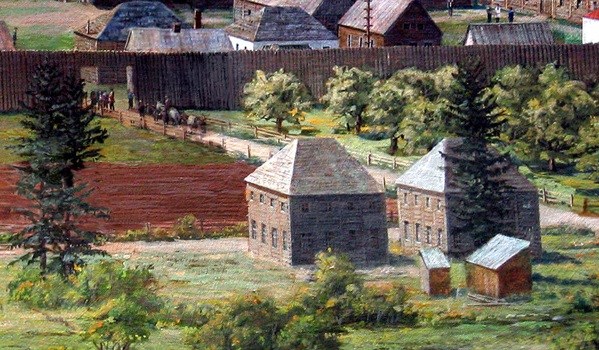The image is a detailed and realistic drawing, depicting a historic settlers' community. It has a rectangular shape, approximately three to four inches wide and three inches tall. The scene portrays two identical two-story brick buildings with sloped roofs that nearly come to a point but instead form a slit. These buildings are positioned side by side, creating a focal point at the bottom portion of the image. Surrounding the buildings, there are various elements that enrich the historical setting. 

In the upper left corner, horses can be seen riding along a dirt path that runs past the buildings and leads to a large wooden fence, taller than the horses, but featuring an opening for passage. Another detail includes the presence of a fortified wall built of trees, enclosing the settlers' homes within a protected, boarded-up camp. The settlement features garden spaces with trees and freshly tilled fields, illustrating the agricultural aspect of the community. 

To the upper right corner, there is a field of trees, while the bottom part of the image is lush with green grass and bushes. Additionally, smaller sheds are located behind the main brick buildings. Throughout the community, people are depicted milling about, engaged in daily activities, further adding to the lively, historical atmosphere of the scene.